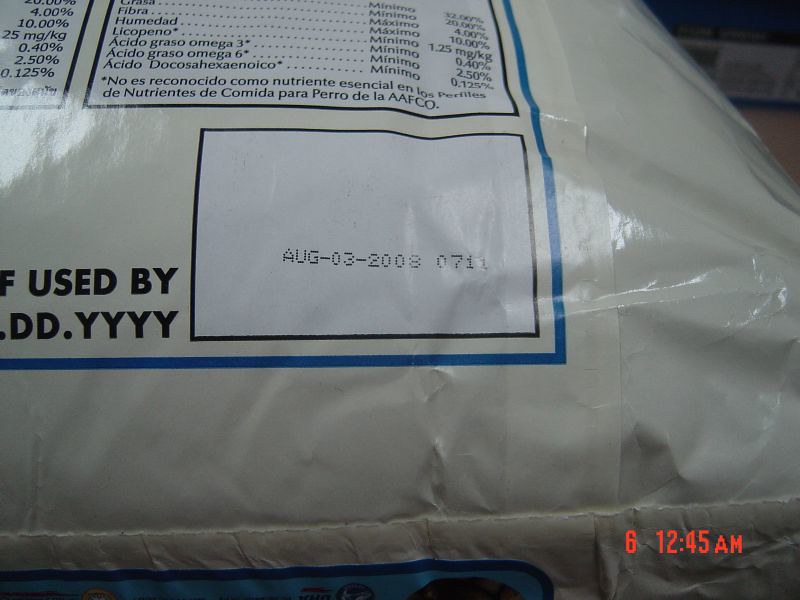Detailed Caption: A white plastic poly bag featuring a distinct blue border can be seen in the image. The bag appears malleable, suggesting it contains a loose substance which could potentially be dog food, a baking ingredient, or fertilizer. Prominently displayed on the bag is a "Best Used By" date of August 3, 2008, situated within a white box bordered in black and red. Additionally, there are sections of text in Spanish, possibly indicating a nutritional or ingredient label, detailed with various percentages. The ingredients list is housed within a separate white box with a black border, making it clearly distinguishable.